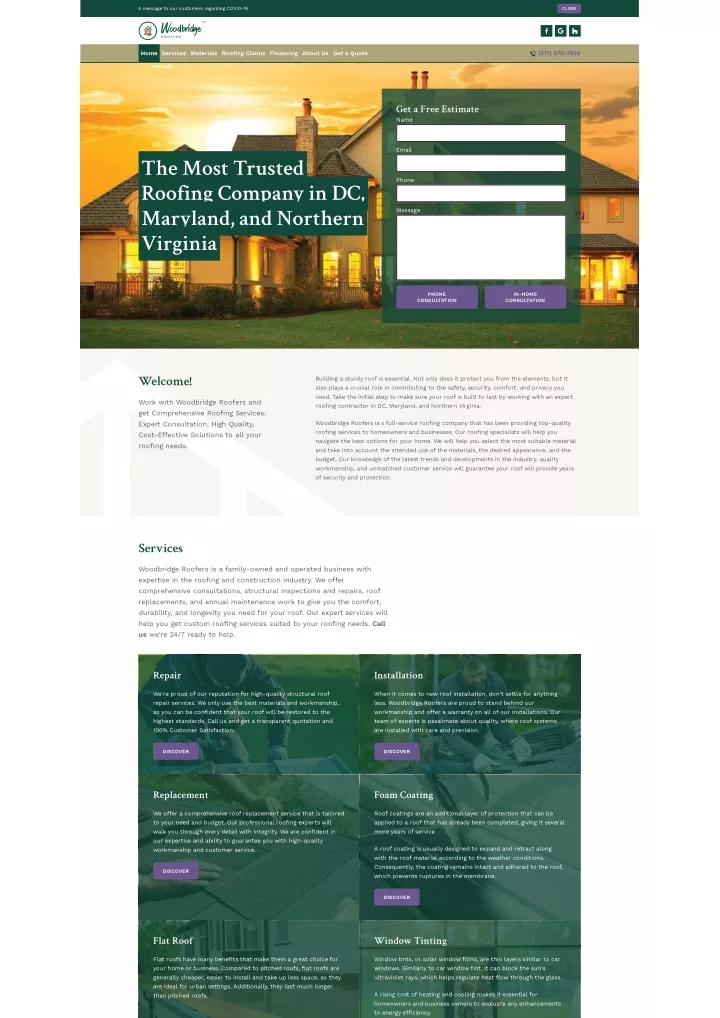The image displays the homepage of the Woodbridge Roofing website, touted as the most trusted roofing company in Washington D.C., Maryland, and Northern Virginia. Dominating the header is a stunning photograph of a large house under an orange-hued sky, indicative of a sunrise or sunset. The house features four chimneys, numerous windows, a well-manicured lawn, and bushes adorning the front yard.

Central to the header is the company's slogan, "The Most Trusted Roofing Company," while to the right, a prominently placed box invites visitors to "Get a Free Estimate." This box contains a form requiring the user's name, email, phone number, and message. Users can choose between a phone consultation or an in-home consultation, submitting their choice via eye-catching purple buttons.

Navigating the site is made easy through a menu bar at the top, featuring tabs for Home, Services, Materials, Roofing Claims, Financing, About Us, and Get a Quote. Below the main header, a welcome message outlines the company's commitment to quality services.

Further down, in green letters, the site highlights its services, emphasizing the durability and longevity of their roofing solutions. This section is divided into four green boxes labeled Repair, Installation, Replacement, and Foam Cutting, each accompanied by a purple "Discover" button. Additional services mentioned include flat roofing and window tinting.